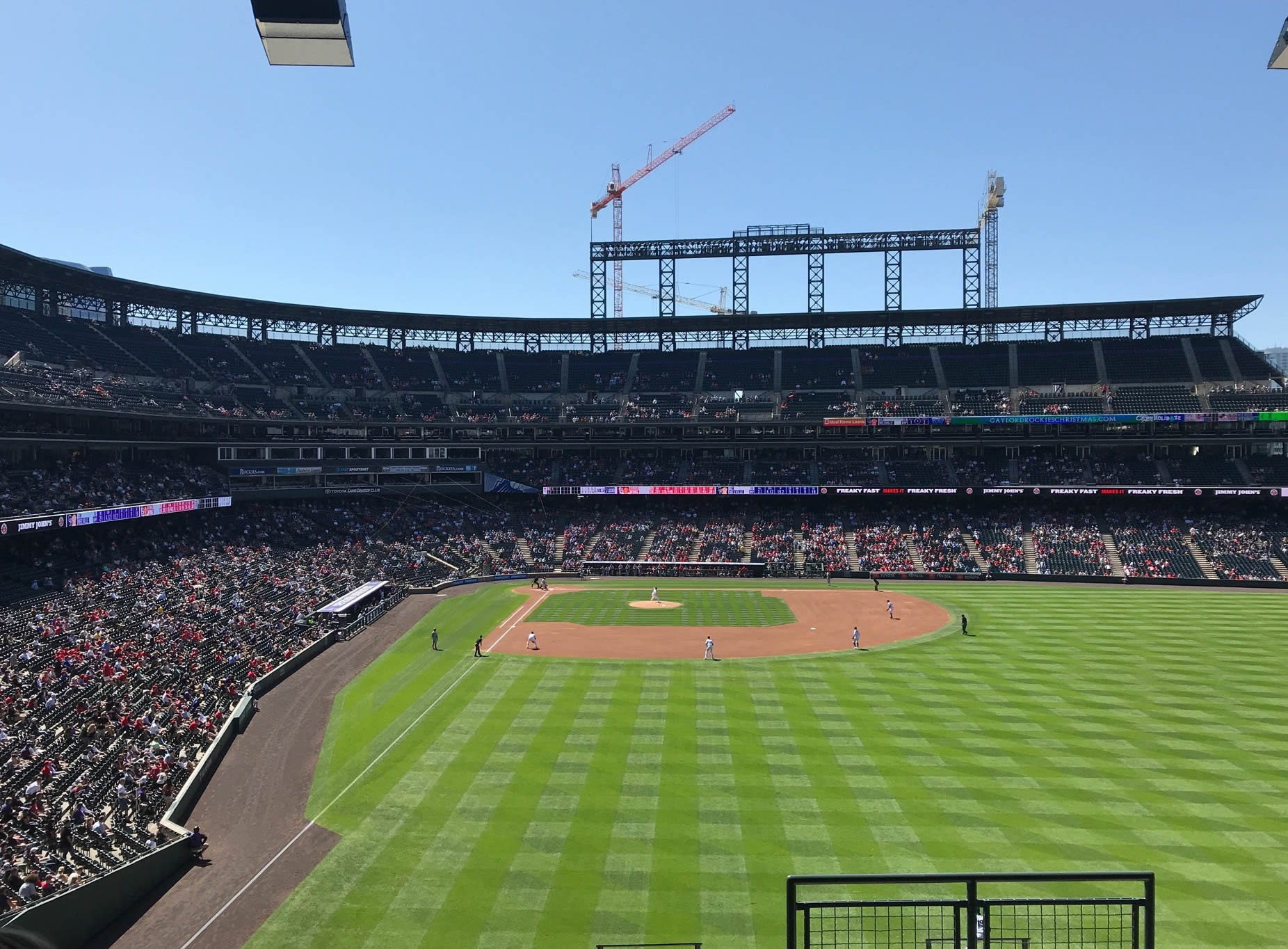In this vivid image taken from the high part of a large, bustling baseball stadium, we see the green expanse of the baseball field, meticulously maintained with a plaid pattern of artificial turf. The bright sun shines down from the left side of the blue, cloudless sky, illuminating the scene below. The stands are packed with spectators, creating a vibrant atmosphere as they watch the game unfold. On the field, the players are primarily positioned on the baseball diamond, with a team on the mound and umpires overseeing the action. Notably, the outfield remains mostly unoccupied, a unique and unusual sight. Surrounding the lush greenery, there is a stretch of gray dirt to the left side, forming a clear boundary. Adding to the dynamic scene, three large cranes are visible beyond the stadium, engaged in construction work. This snapshot captures a lively game day, the sun casting a radiant glow over the entire stadium.